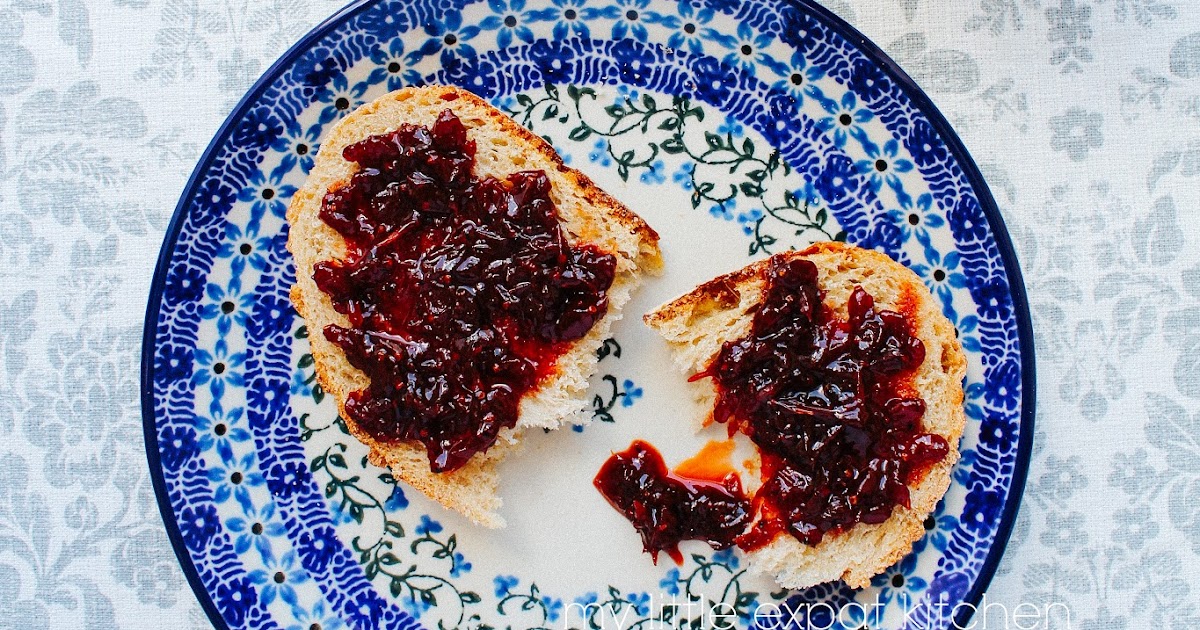This overhead photograph features a classic antique white plate adorned with intricately designed blue floral patterns and a dark blue border composed of three distinct lines. The plate has a white center embellished with delicate green vines and light blue flowers. Positioned on this decorative plate is a piece of toasted, oval-shaped French bread split into two halves, with a generous spread of dark-colored berry jam, possibly cherry or raspberry, on each half. A small smear of jam can also be seen on the plate itself. The plate rests on a damask tablecloth featuring an elegant blue and white floral pattern, complementing the ornate design of the plate.